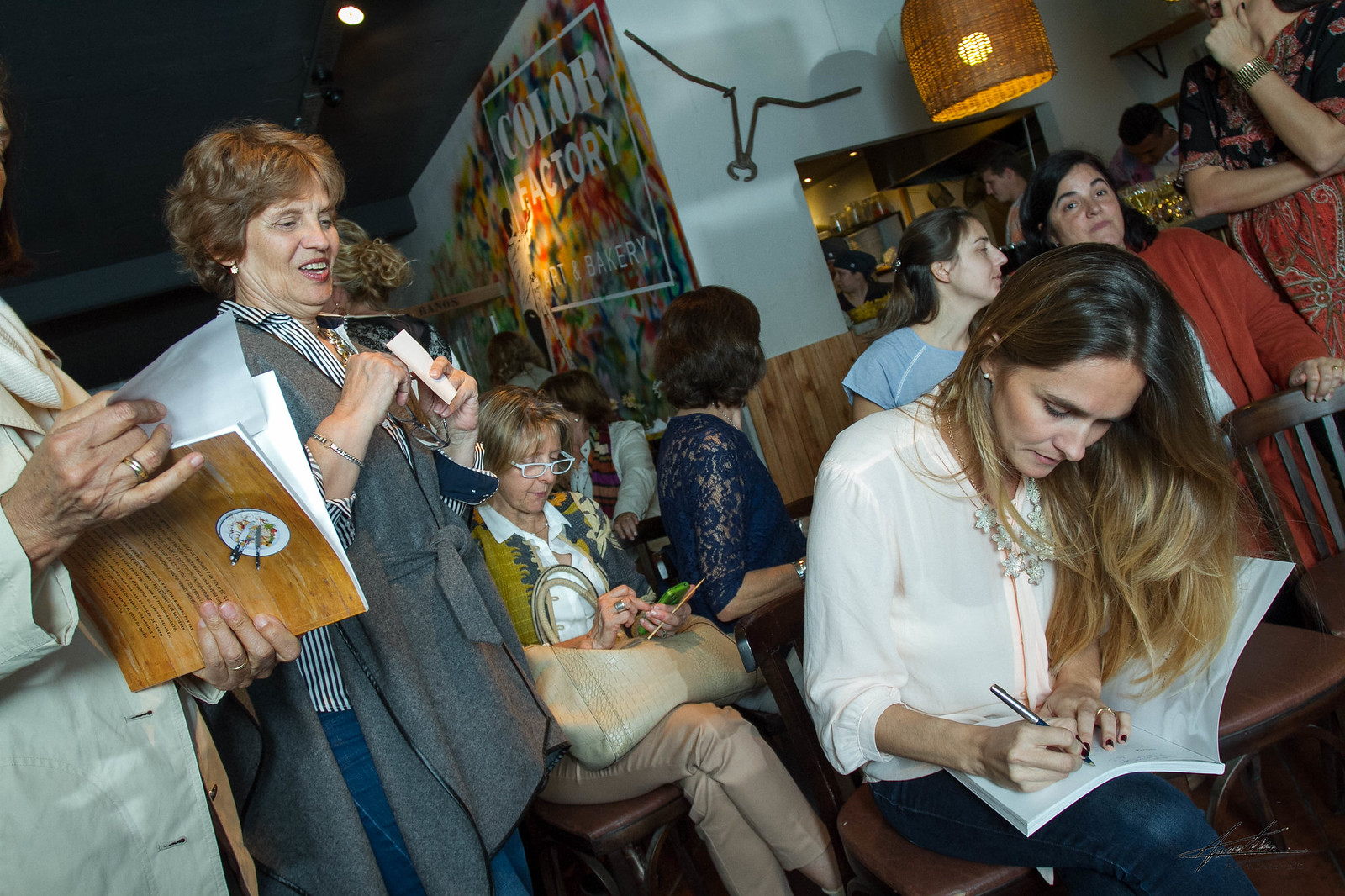The image captures a bustling scene inside the Color Factory, Art, and Bakery, where a book signing event for a female author is taking place. The landscape-oriented color photograph showcases a lively atmosphere with numerous women engaged in various activities. In the immediate foreground, a woman with long brown hair in a pink blouse and a ring on her left hand is signing a book with a dark-painted ink pen. The book she is signing has white pages. Surrounding her, several females can be seen either standing or sitting, engaging in conversations or waiting patiently in line for their turn to get their books signed. To the left, a woman in white glasses and a gray jacket, holding a phone and smiling, sits with a purse in her lap. Another woman nearby, wearing a cream-colored jacket and rings on both hands, holds an open book. Further to the right, a woman in a white shirt and blue jeans, seated and facing the corner, is making notes in an open workbook with a silver pen. Beyond this, the background buzzes with mingling groups of women, some seated in wooden chairs, under a partially visible sign reading "Color Factory, Art, and Bakery." The overall scene captures the vibrant and communal spirit of the event with women connecting and interacting in a cozy, artistic setting.